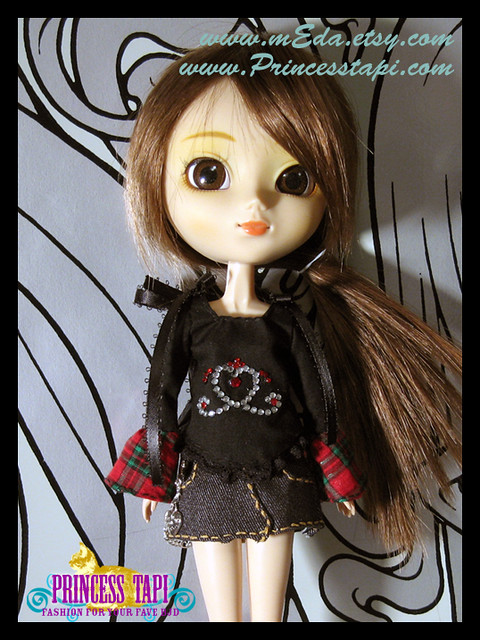This detailed image features a charming doll prominently displayed against a gray and white, swirled background pattern. In the top right corner, the URLs "www.meda.xc.com" and "www.princesszapi.com" are visible. The doll itself is characterized by its large, round head with long dark brown hair styled into a ponytail that drapes to the right. She has strikingly big brown eyes and a fair complexion. The doll is dressed in a black sweatshirt adorned with a jewel-encrusted heart, paired with a denim skirt. Adding to her ensemble, she has red and green plaid armbands. The bottom left corner features the name "Princess Toppy," written in pink, followed by the phrase "Fashion for your fave UJD" also in pink. There is also a golden cat subtly placed in the background.